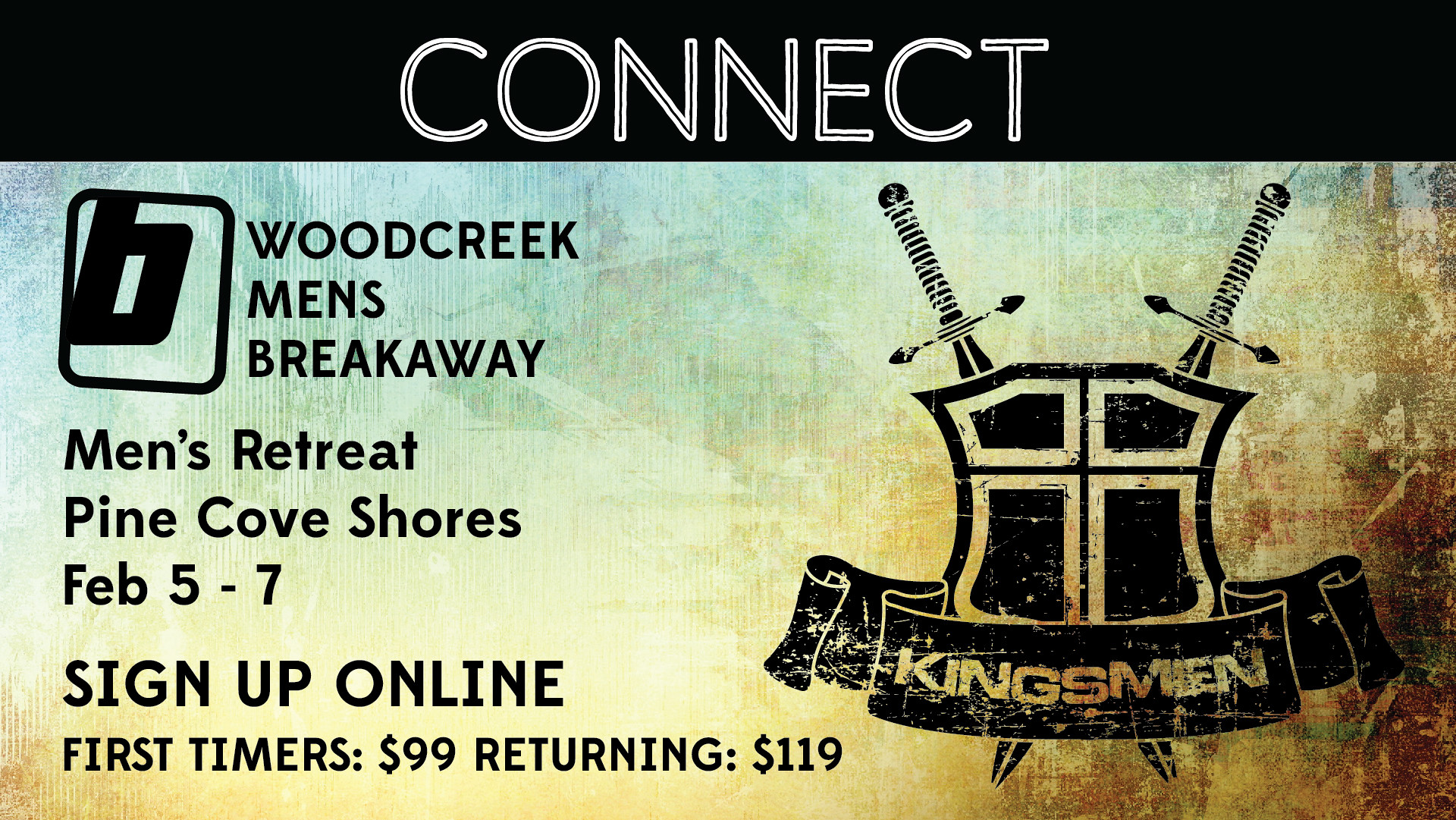The image is a digitally synthesized advertisement poster with a textured background that fades from dark brown in the bottom right corner to lighter yellow, then to a bluish-green in the top left corner. Across the top of the image is a black bar with the word "CONNECT" in large white capital letters centered within it. Below this, on the left side of the image, the text "WOOD CREEK MEN'S BREAKAWAY" is written in black capital letters. Adjacent to this text is a logo featuring a lowercase 'b' inside a rounded black box outline. Beneath the logo and the heading are the details "MEN'S RETREAT PINE COVE SHORES, FEB 5 TO 7. SIGN UP ONLINE," all in capitals, followed by "First timers, $99; returning $119." On the right side of the image, there is a stylized black cartoon shield with two crisscrossing swords behind it. Overlaid on the shield and swords is a banner with the word "KINGSMEN" written across it. The imagery evokes a coat of arms and is depicted in a clip-art style.